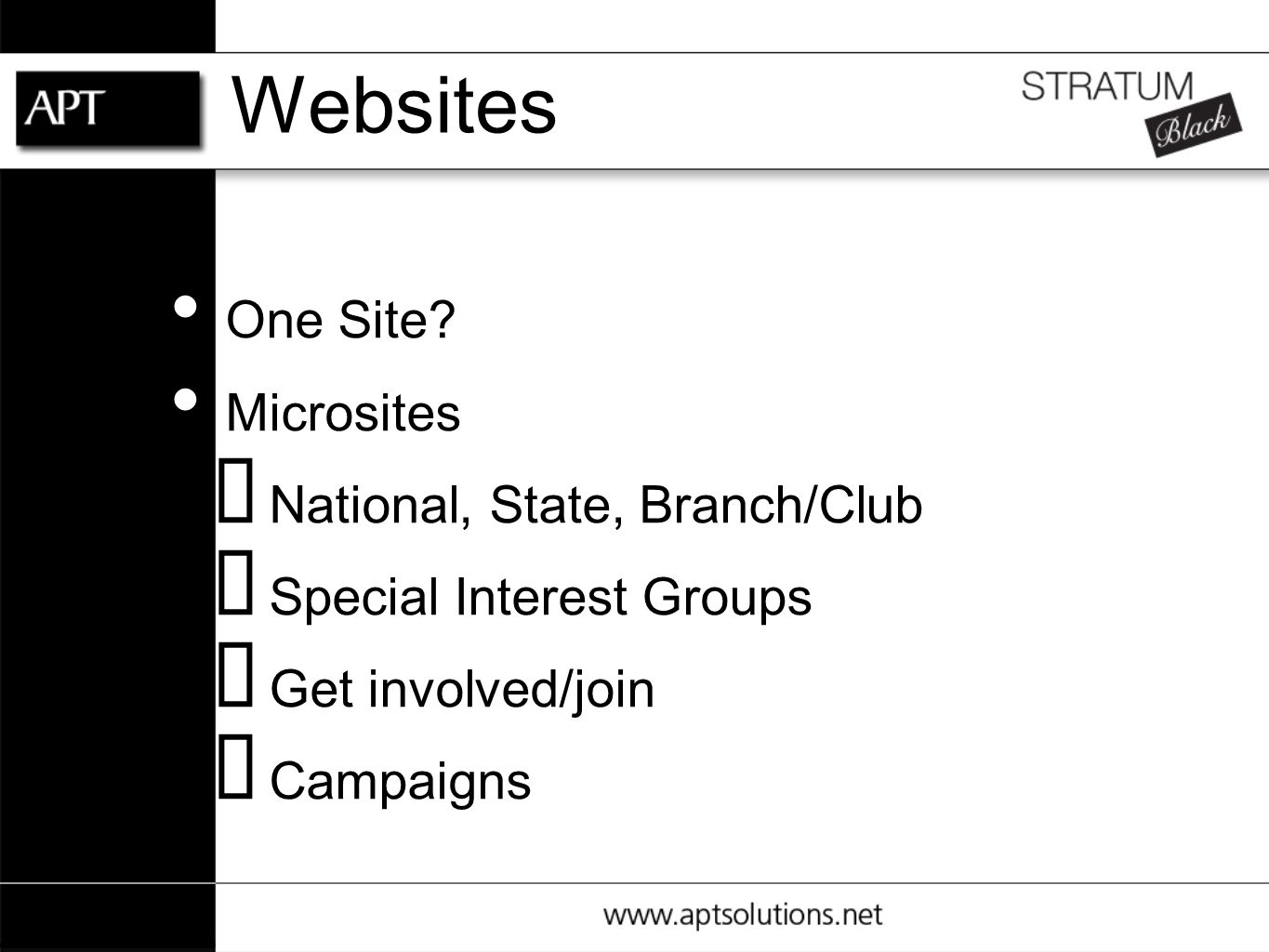The image is a black-and-white advertisement that resembles a Microsoft PowerPoint slide with a modern, minimalistic design. On the left side, there is a vertical solid black bar serving as a border. At the top of the image, a horizontal white bar spans across with the letters "APT" in black text, providing a distinct header against the black background. To the right of this bar, the words "Websites Stratum Black" appear in a structured format, with "Black" in cursive script.

Beneath this white bar, a list of bullet-point items is displayed, aligned next to the black vertical bar on the left. The items read as follows:

1. One Site
2. Micro Sites
3. National/State/Branch/Club (preceded by an empty square)
4. Special Interest Groups (preceded by an empty square)
5. Get Involved/Join (preceded by an empty square)
6. Campaigns (preceded by an empty square)

At the bottom of the list, the URL "www.aptsolutions.net" is provided. The overall style is streamlined, focusing solely on black and white text with minimal graphical elements.